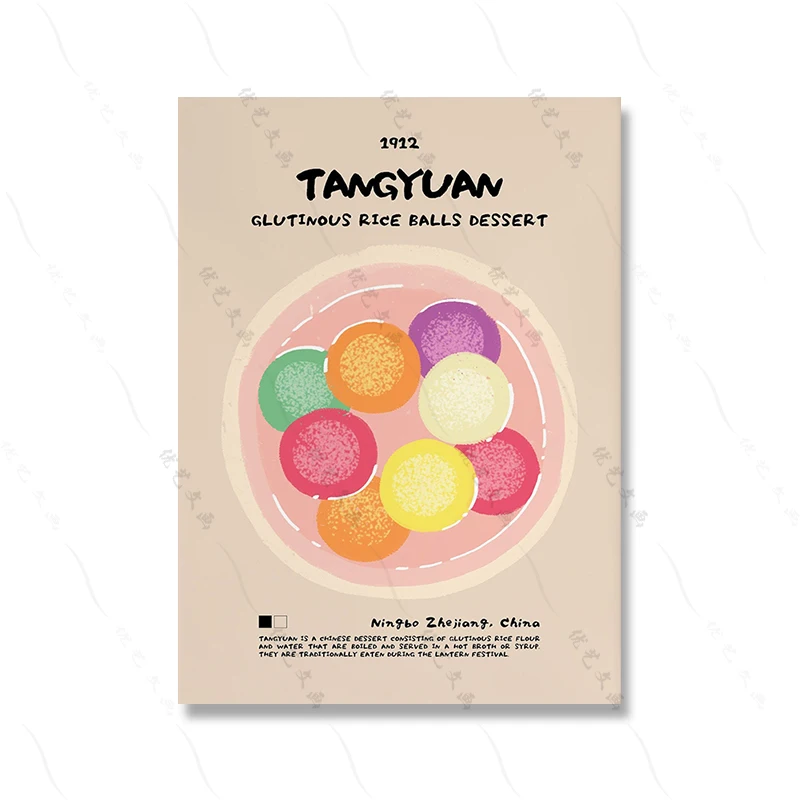The image likely represents an illustration that resembles a book cover, crafted from beige paper. The illustration prominently features a pink bowl filled with various colored balls, specifically orange, pink, green, purple, and yellow. At the top of the image, "1912" is inscribed in black lettering. Below this date, the title "Tangyuan" appears, followed by the phonetic spelling "T-A-N-G-Y-U-A-N." The subtitle reads "Glutinous Rice Balls Dessert." Further down, the text "Mingzhou, Zhejiang, China" is displayed. The description beneath the illustration explains that Tangyuan is a traditional Chinese dessert made from glutinous rice flour and water, which is boiled and typically served in a hot broth or syrup. This dessert is traditionally consumed during the Lantern Festival. Overall, the flat appearance of the image makes it ambiguous whether this is an actual book cover or simply an artistic illustration designed to resemble one.